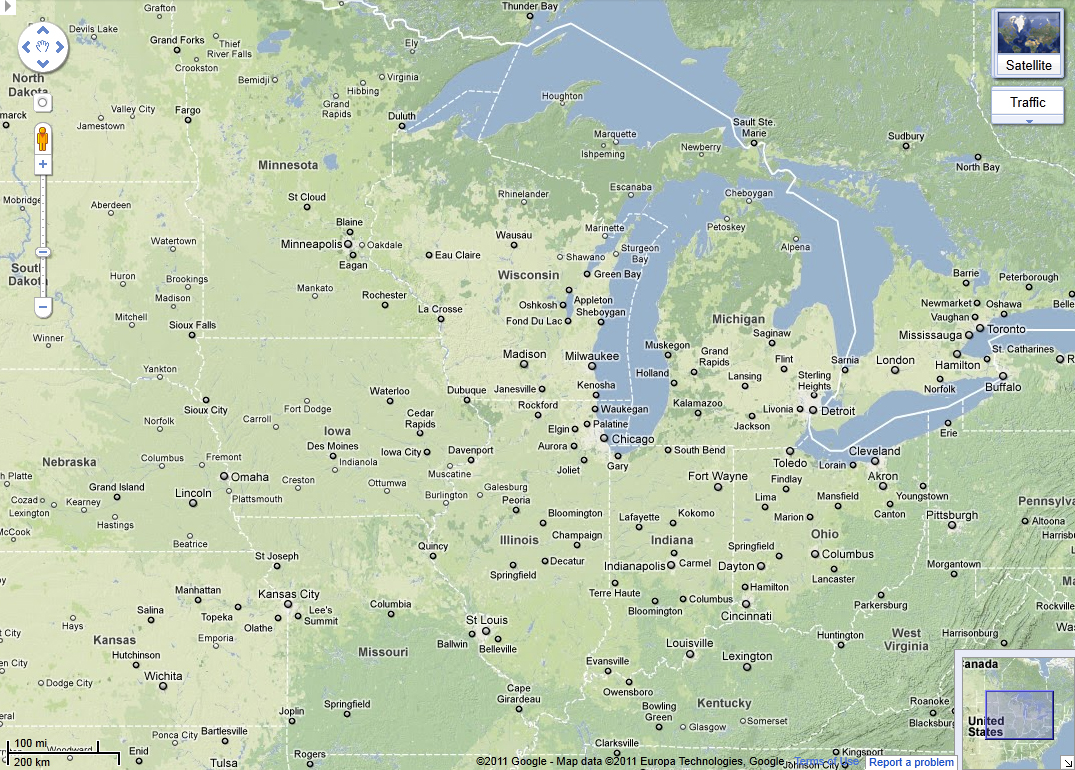This image is a detailed satellite map of the central United States, featuring various states and prominent cities. In the upper right-hand corner, the Great Lakes are visible, showcasing their vast expanse. Kansas City, located in Kansas, is positioned in the lower left-hand corner of the image. The map also highlights the state of Nebraska, with the landscape depicted in varying shades of green, indicating different types of terrain and vegetation.

Numerous towns and cities are labeled throughout the map, providing a comprehensive view of this region. Key locations include Frankfort, Illinois, and St. Louis, as well as Rochester and Minneapolis, Minnesota. Further north, the cities of Grand Forks and Fargo are noted. The details suggest that this map was captured from a computer screenshot, indicated by its high-resolution and the clear demarcation of urban and rural areas.